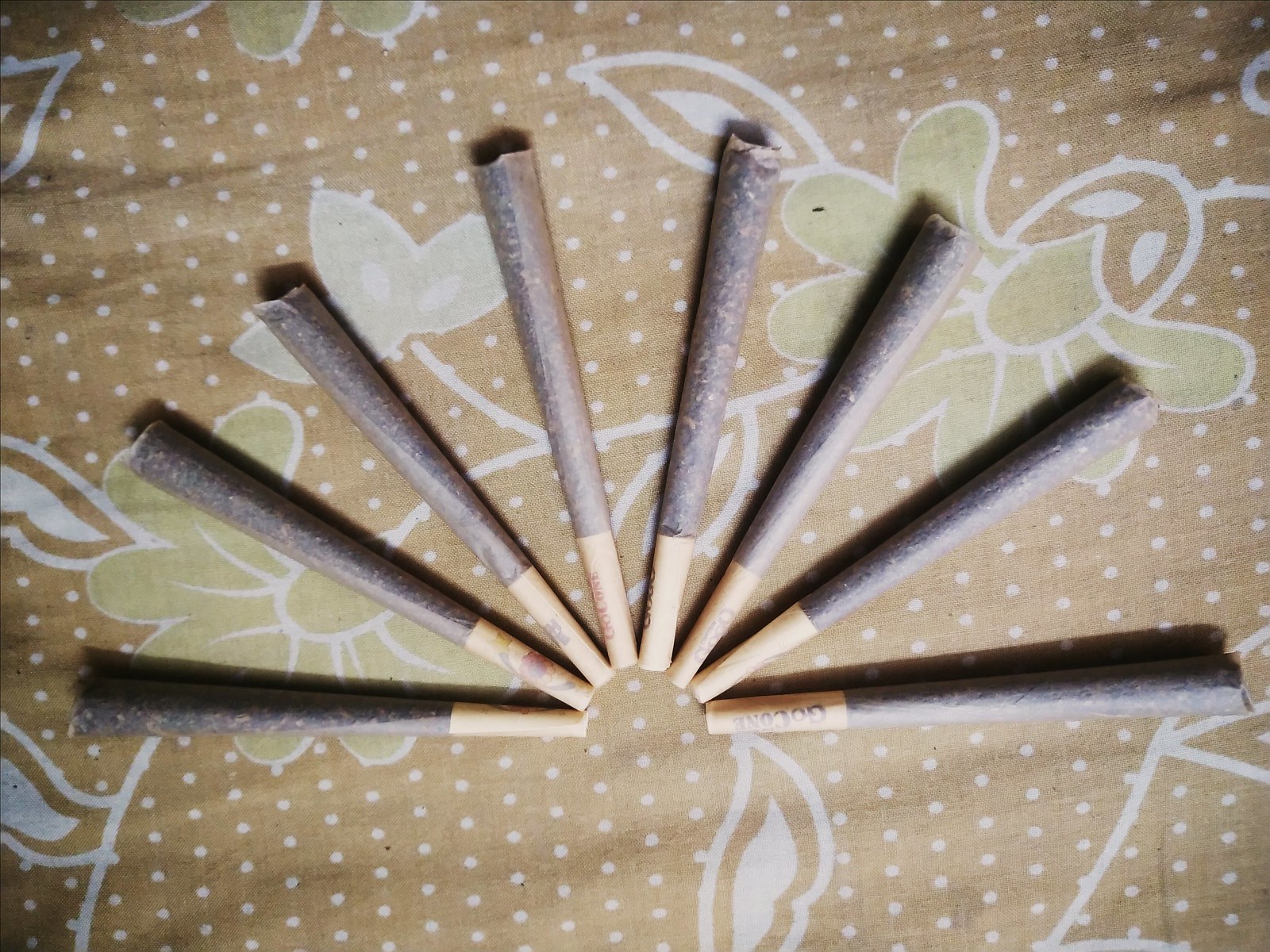The image depicts eight hand-rolled cigars or cigarettes, arranged in a fan-like, semicircular formation. Each item transitions from a thinner light brown, possibly filtered, tip to a thicker, darker brown rolled side, showcasing visible seams and edges. They are meticulously placed with their tips touching, forming a cohesive pattern reminiscent of a flower. This setup sits on a tan-colored fabric, adorned with white polka dots and green floral designs, including white leaves and stems that interconnect, contributing to the overall aesthetic. Wrinkles and folds in the fabric add texture to the scene, accentuating the carefully curated arrangement of the cigars.